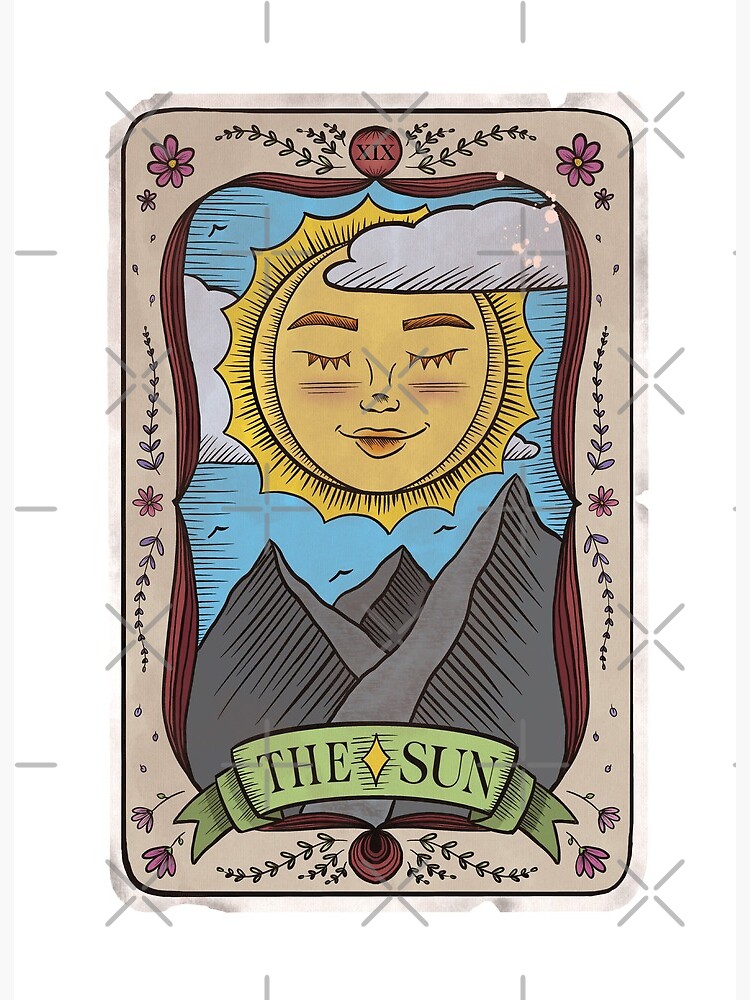This image features a close-up of a tarot-like card with a creamy beige background and rounded corners. The card is centered against a white backdrop patterned with a repeating watermark composed of Xs with gaps and plus signs missing their centers, arranged in alternating rows. The card itself has a white border framed by a thin black line, containing detailed illustrations.

At the top of the card is a brown balloon shape with the Roman numeral "XIX" inside. The central image depicts a whimsical sun with closed eyes adorned with eyelashes, eyebrows, blush on its cheeks, and lips, creating a serene, human-like expression. The sun floats in a blue sky dotted with two white clouds and several simplistic birds soaring above a trio of gray mountains.

Encompassing the card’s central scene are various sketches of flowers and leaves. Purple and pink flowers with yellow centers and green stems decorate all four corners and along the sides, contributing to the card's intricate border design. At the bottom, a green banner emblazoned with "The Sun" in black letters, separated by a yellow diamond, completes the card's motif. The overall appearance of the card is striking, with vibrant yet vintage colors adding to its mystical and aged charm.